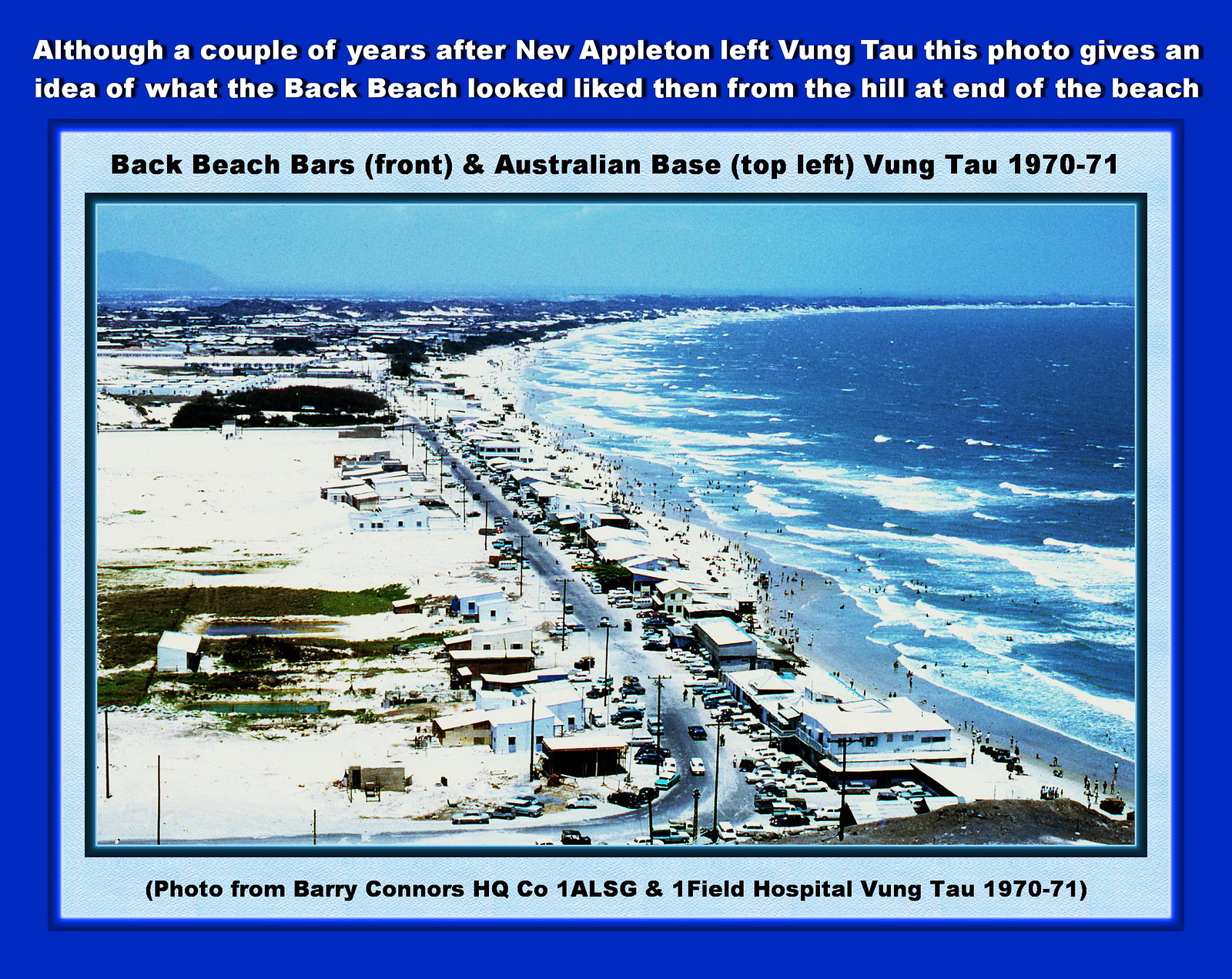This image depicts the back beach of Vung Tau circa 1970-71 from a vantage point on the hill at the end of the beach. Enclosed within a blue border, the photograph features descriptive text in white font above it, stating: "Although a couple of years after Nev Appleton left Vung Tau, this photo gives an idea of what the back beach looked like from then from the hill at end of the beach." In black font above the image, it reads: "Back Beach Bars front and Australian base top left Vung Tau 1970 to 71." Below the image, it says: "Photo from Barry Connors HQ CO 1 ALSG and 1 Field Hospital Vung Tau 1970 to 71."

Within the image, the ocean stretches along the right side, meeting the shoreline that runs diagonally from the bottom right to the upper left corner. The sandy beach is populated with people both on the shore and in the water. A road runs parallel to the beach behind a row of houses and bars. Further inland, there are clusters of additional houses and buildings, accompanied by green patches. The background features hazy blue skies with a couple of mountains. The scene includes cars parked along the road, highlighting the settlement's activity. Streetlights line the area near the buildings, providing additional details to this snapshot of Vung Tau's back beach during that period.